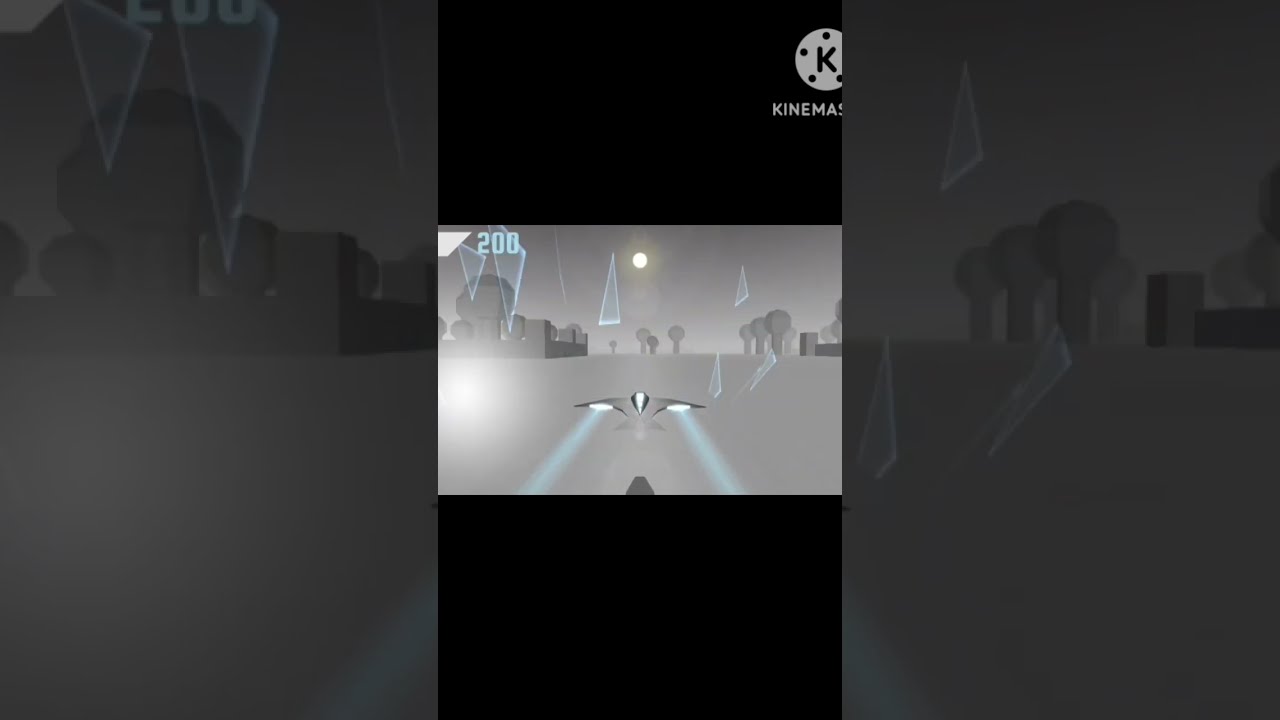This image is a screen grab of a video game featuring a sleek, bird-shaped airplane with jet propulsion coming out of its wings, centered in the middle of the scene. The game environment appears to be a grayscale, possibly alien landscape with block-like structures and digital trees that lack distinct leaves or branches. The airplane is flying towards a backdrop dominated by a bright yellow sun in the top center, contrasting with the overall gray tone of the image. Scattered around the plane are translucent blue, sharp, triangle-shaped objects. In the top right corner of the image, there is a partially cut-off logo that reads "Keen MA" or "kind master" in white text, centered within a white circle featuring a black 'K'. The scene evokes a simplistic, almost Minecraft-like graphical style and suggests a flying game with basic yet vivid digital elements.